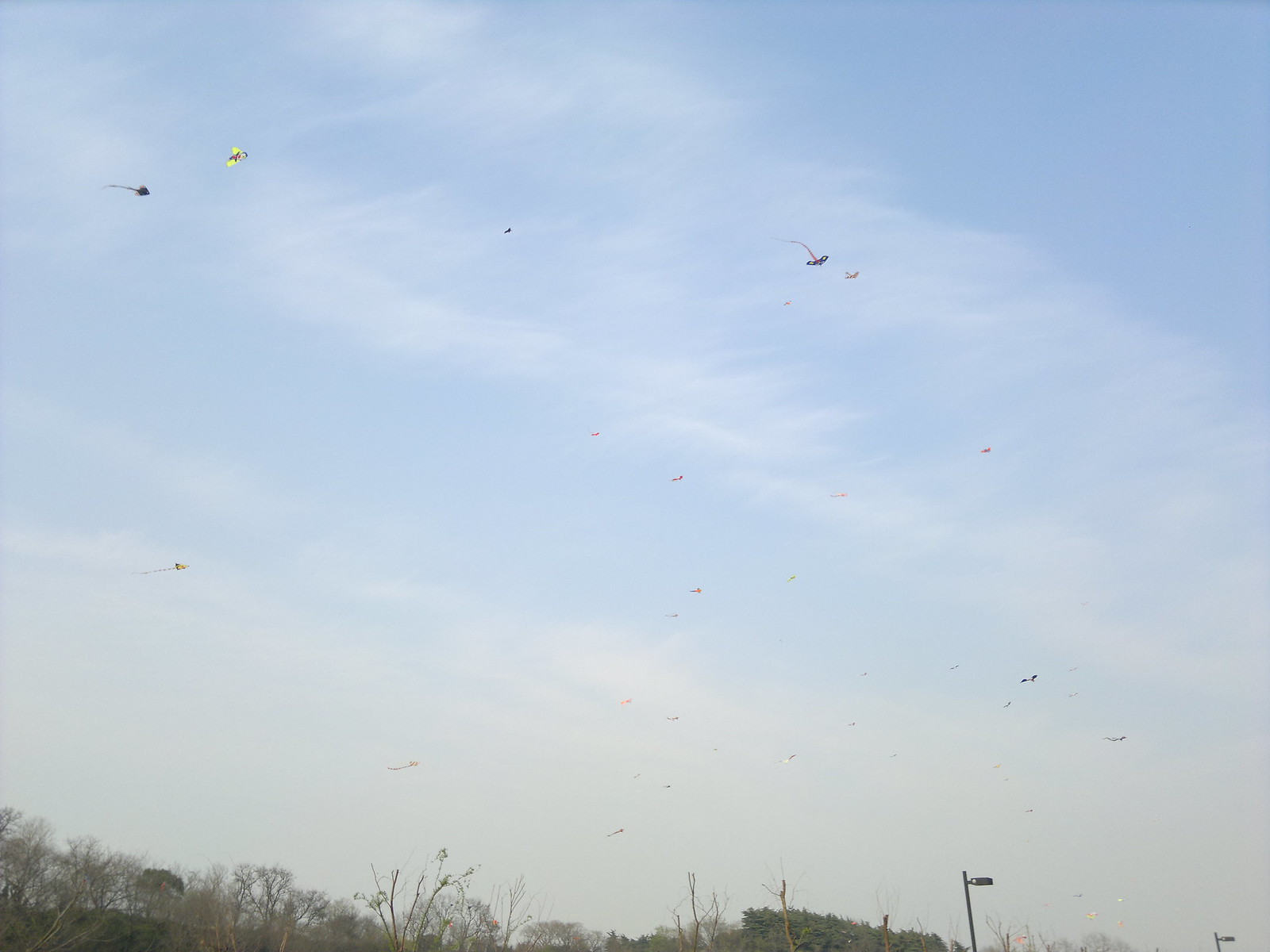The image captures a serene outdoor scene dominated by a vast, light blue sky adorned with scattered, whispery white clouds. The horizon is lined with gently rolling hills, populated by a mix of trees. Some trees stand bare, while others cling to the last of their leaves, hinting at the cusp of winter. Among them, resilient evergreen and pine trees maintain their dense, green foliage. A brown metal pole of a street light rises from the ground, anchoring the scene.

Hovering in the sky are numerous kites—some soaring high, others lower, with varying sizes. A few kites trail long, playful tails, while others remain tail-less. Though small and scattered, the kites are distinguishable, with at least one featuring a vibrant highlighter-yellow hue. The kites pepper the sky, almost reminiscent of a flock of birds, adding a dynamic element to the otherwise tranquil landscape.